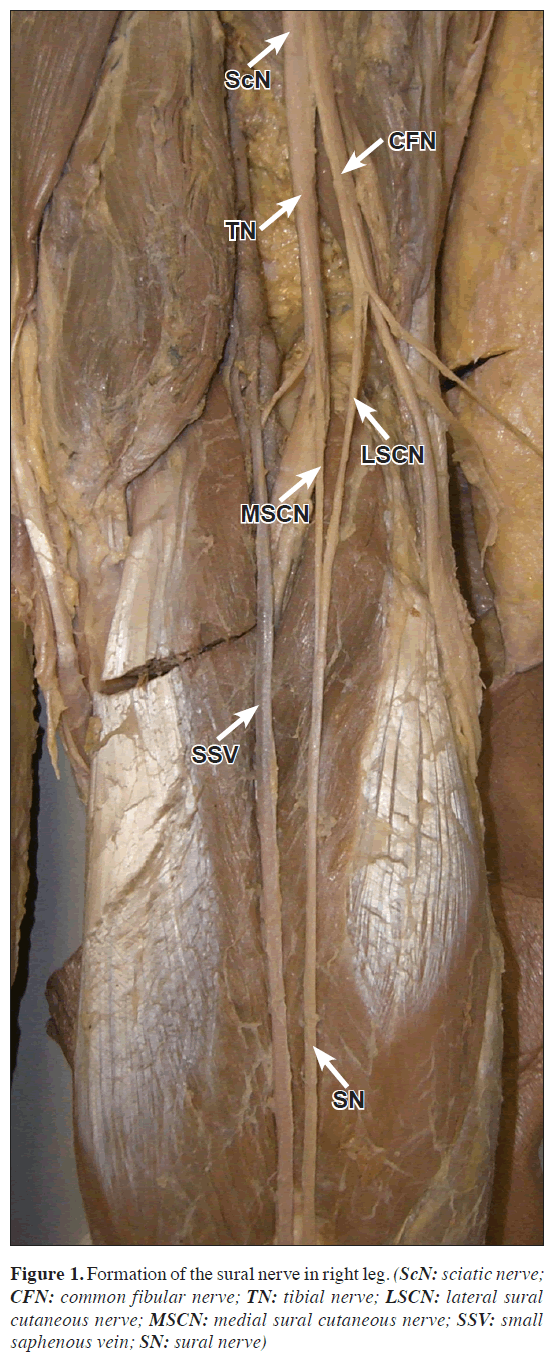This image, taken from a medical educational setting, illustrates the formation of the sural nerve in the right leg. Comprised of various shades of brown, white, and black, the photograph appears to depict a dissected or digitally rendered view of leg muscles, veins, and nerves, shown in a narrow rectangular format. The nerves, labeled with black abbreviations, include SCN (sciatic nerve), CFN (common fibular nerve), TN (tibial nerve), LSCN (lateral sural cutaneous nerve), MSCN (medial sural cutaneous nerve), SSV (small saphenous vein), and SN (sural nerve). White arrows point to these specific nerve structures on the brown, textured background. The text "Figure 1, Formation of the Sural Nerve in the Right Leg" is printed at the bottom of the image, along with these labels, providing detailed anatomical information aimed at a medical audience.